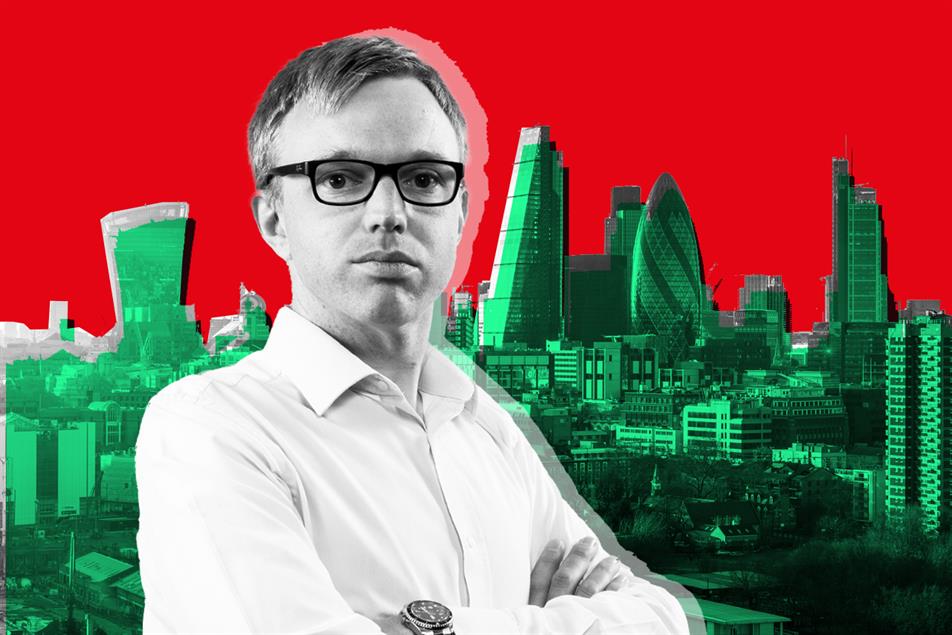In this striking photo, a young man is captured in black and white, positioned slightly to the left of center, with his face and part of his upper body clearly visible. He stands with his arms crossed in front of him, wearing a white, collared, button-up shirt and a wristwatch on one hand. His light-colored hair is short and swept to the front, and he sports black-rimmed glasses. His expression is somewhat smug, with big eyes spaced far apart and a mouth closed in a neutral line. The background presents a vibrant contrast, depicting a cityscape with densely packed, green-tinted skyscrapers and tall buildings. Above this urban jungle, the sky is a vivid, candy apple red, creating a visually arresting red and green filter effect against the monochrome figure in the foreground.